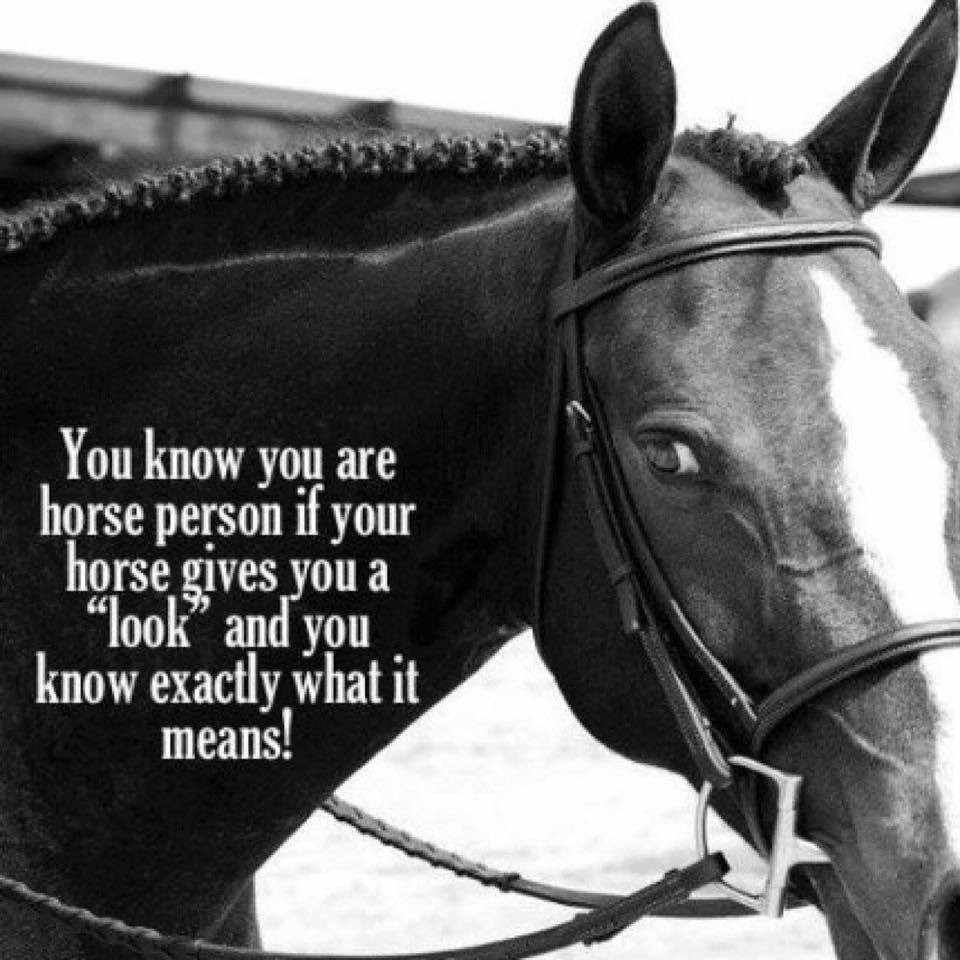This is a detailed black-and-white photograph of a dark-colored horse taken from the side, showcasing its head and neck. The horse's gazing eye and pointed ears suggest it's looking slightly behind and off to the side. Notably, the horse has a white stripe running down its forehead to its muzzle, contrasting with its dark mane, which is intricately braided into small knots. The horse is equipped with a bridle and a bit in its mouth. Over the image, white text digitally added reads: "You know you are a horse person if your horse gives you the look and you know exactly what it means." The caption, with a hint of humor, aims to resonate with horse enthusiasts.